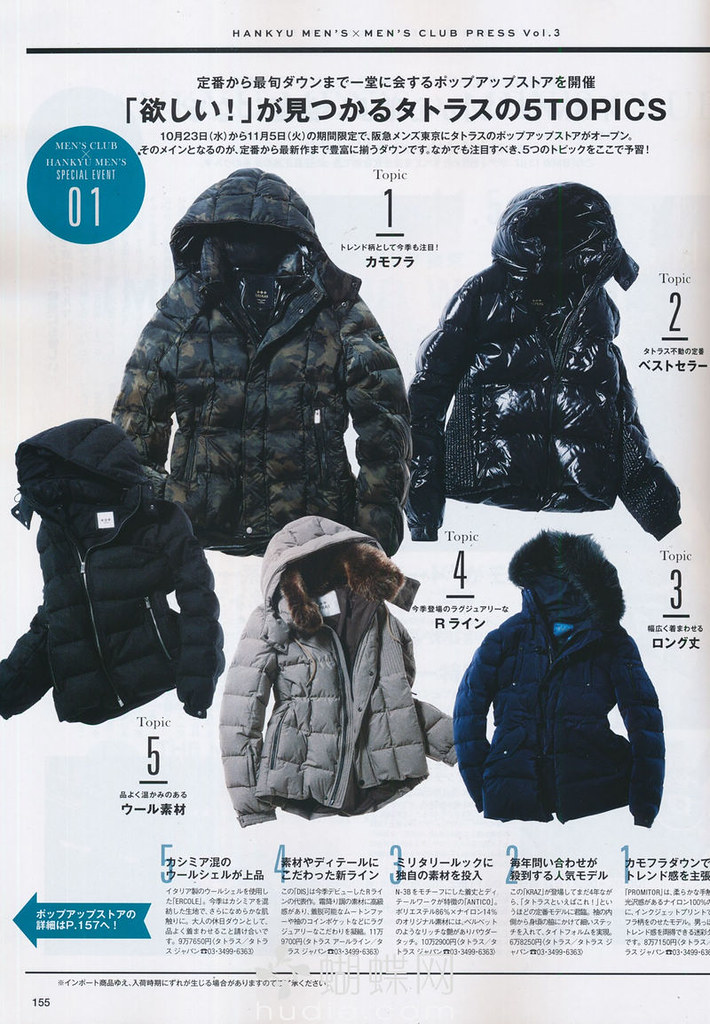This image appears to be a scan or photograph from an Asian magazine, featuring an advertisement for heavy winter coats. Across the top, in English, the text reads "Han Kyu Men's X Men's Club Press Volume 3," followed by several lines of Asian script. The page is divided into two sections: the upper half displays two black jackets with hoods on either side, with the left one being made from a less shiny material compared to the shiny vinyl or plastic-looking one on the right. The lower half showcases three more jackets: a camouflaged one, a light gray puffy one, and a dark blue corduroy jacket with fur around the hood. Each coat is numbered from one to five, with associated Asian text below. Additional features include a blue circle at the top left marked '01' in white and a blue arrow with more white text in the bottom left corner. The background splits into light gray and white.